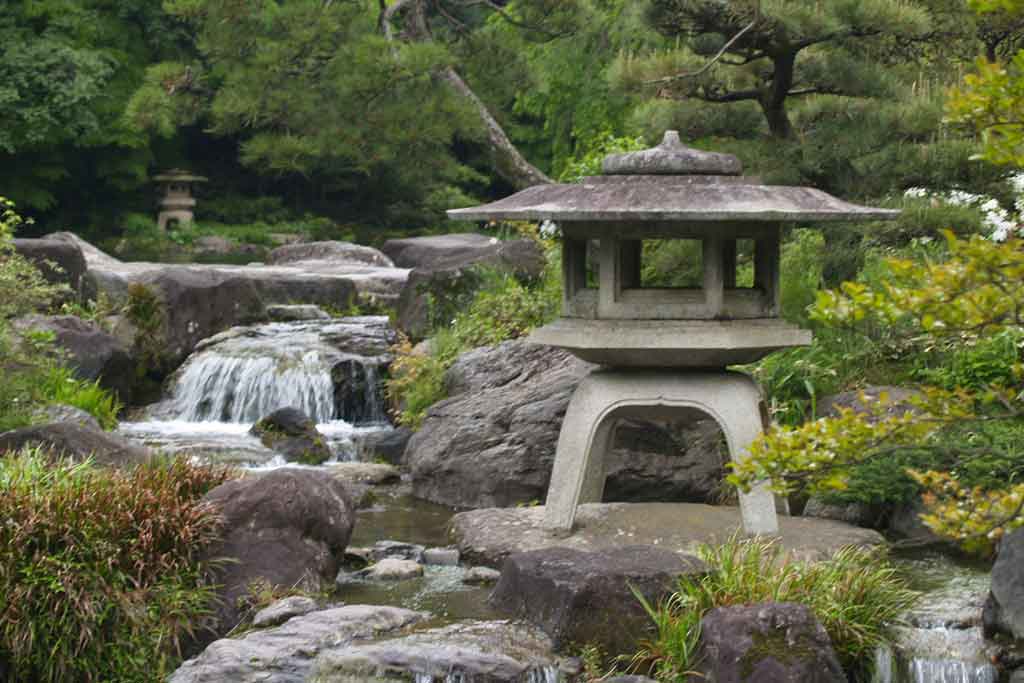This photograph captures a serene garden, likely located in Asia, featuring a picturesque stream cascading over rocks, forming a couple of small waterfalls. The scene is rich with greenery, including trees, wild brush, and deciduous plants interspersed among the gray rocks. Centrally and notably within the stream, there is a distinctive stone structure resembling a miniature pagoda. This intricate structure, which boasts openings in its sides and a circular roof, is perched on a round stone in the middle of the flowing water. It rests atop a simple, plastic-like step stool, giving the impression of a decorative element purposefully positioned in the natural setting. Another similar stone pagoda can be seen in the distance to the back left. The image was taken during daylight on an overcast day, encapsulating the tranquil ambiance of this outdoor garden space.